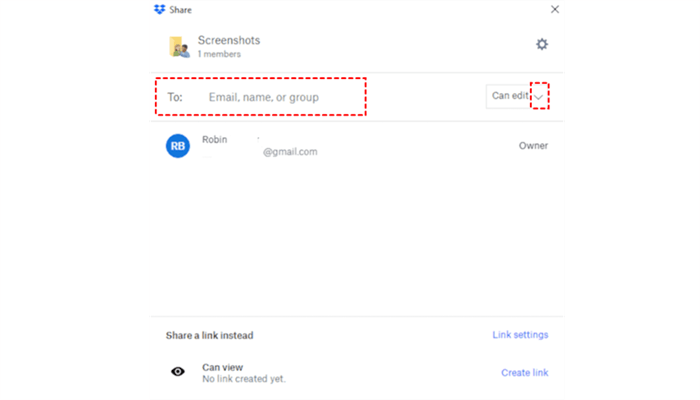The image appears to be a screenshot of a sharing interface, likely from a file or document sharing service. At the top of the interface, there is a 'Share' option, identifiable by a blue tool icon. In the top-right corner, there's an 'X' to close the sharing window.

Below this, the section labeled 'Screenshots' indicates one member is currently viewing or has access. Adjacent to the section titled 'Screenshots' is an icon resembling a door with two people standing next to it. The two figures are of different skin tones, one fair-skinned and the other darker-skinned, though their gender is indistinguishable.

Further down, there's a portion bordered by red perforated dots, displaying the number '2', followed by fields labeled 'Email', 'Name', and 'Group'. To the right of these fields, there’s an option indicating 'can edit', with a checkmark beside it. This checkmark also has a red perforated outline, suggesting it might be part of a dropdown menu.

Below this, an 'RB' icon appears, annotated with the name 'Robin', who is identified as a Gmail owner. There's also an instructional message: 'Share a link instead', next to an 'I' symbol and the note 'can view, no link created yet'. On the right side, buttons for 'Link settings' and 'Create link' are visible.